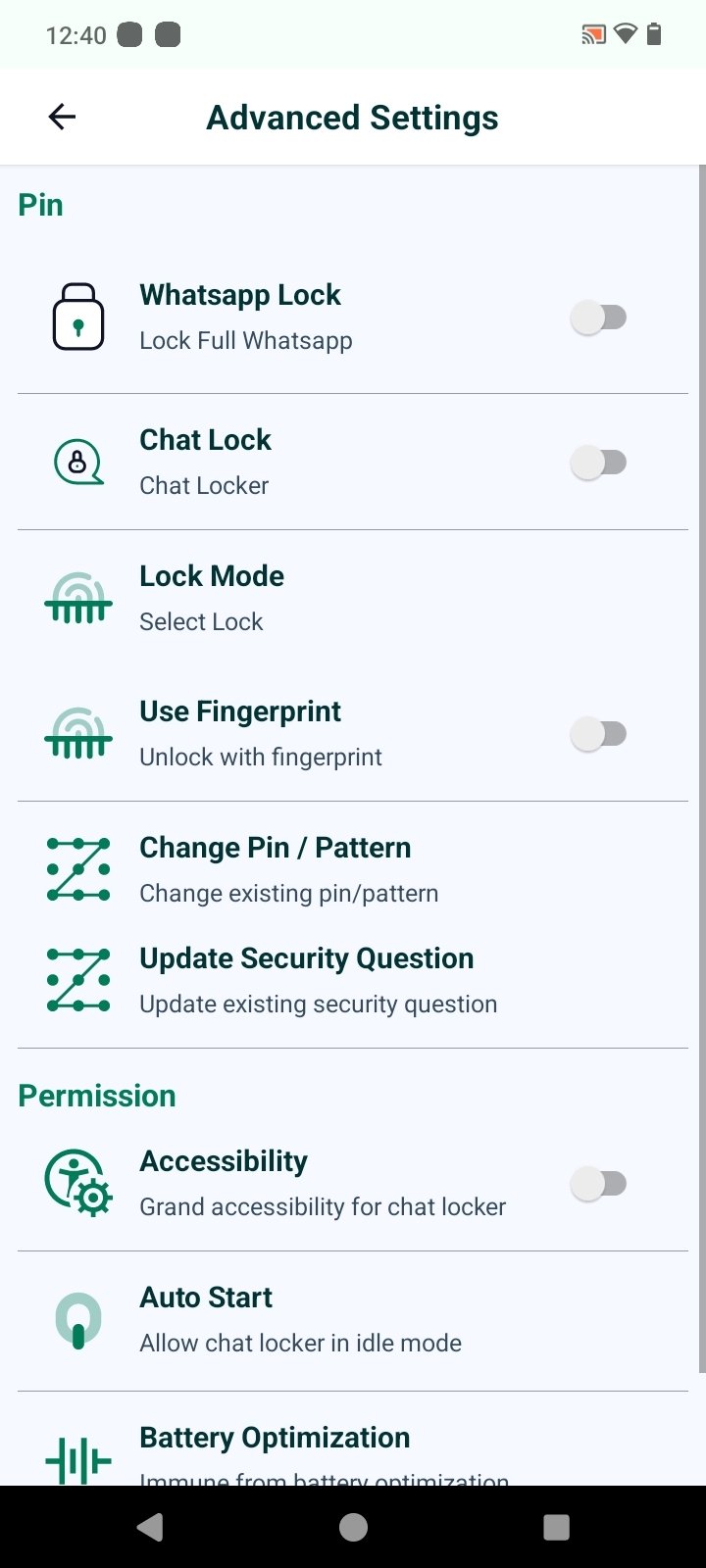The image features a user interface predominantly set against a white background. At the top, there is a light gray box containing red text with an arrow pointing left, labeled "Autoresponder." Below this box, a text field includes a phone icon. Adjacent to it is a circle with a question mark, followed by a settings icon depicting a gear.

Continuing down, a white box with a gray border hosts the label "Contact Settings." Inside this box are four horizontal lines, each paired with a blue circular checkbox. The top checkbox is selected, filled in dark blue, while the others remain unselected. The text labels next to the checkboxes read, from top to bottom: "Everyone," "My Contact List," "Except My Contact List," and "Except My Phone Contact."

Further below, another white box with a gray border is labeled "Contact List." This box includes a dark green circle with two diagonal arrows. Beneath this symbol, the text reads "Auto Reply to Everyone."